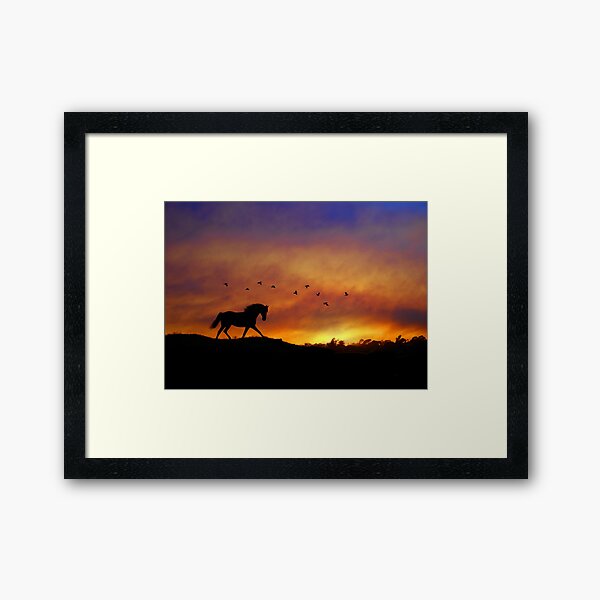The image showcases a photograph of a painting centered on an off-white wall. The painting, encased in a sleek black wooden frame with a thick border, also features an inner off-white matting. Dominating the composition, the painting vividly captures a twilight scene where a silhouetted horse, in mid-gallop, charges towards the right across darkened grass. Above the horse, about ten black birds dot the evening sky. The sky itself transitions mesmerizingly from deep blue at the top through layers of light gray, to orange, brown, and finally pale yellow hues at the horizon, indicating the sun has just set. Subtle curves in the landscape add a dynamic sense of movement, complementing the energetic posture of the horse.